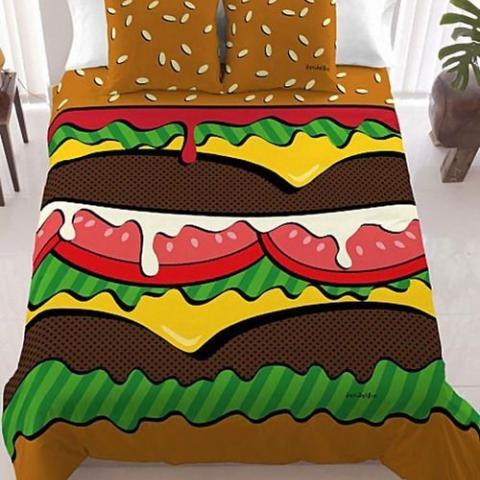This image showcases a unique and detailed hamburger-themed bed set, vividly designed to resemble a fully stacked hamburger. The bedspread mimics the layers of a burger, starting from the top with what appears to be a sesame seed bun cover, characterized by its rusty brown color and white sesame seed patterns on the two top pillows, imparting a realistic touch. The visual delight continues with a cascade of vibrant hamburger dressings: a layer of red ketchup or tomato slices drips beneath the bun, followed by lush green lettuce. Below this, a slice of yellow cheese rests atop a juicy brown hamburger patty.

The intricate design does not stop there; a subsequent tier introduces a creamy layer of white mayonnaise mixed with tomatoes, followed by more green lettuce, another slice of cheese, and a second brown hamburger patty. Finishing this culinary creation is another layer of green lettuce leading to the bottom bun, completing the look of a perfectly assembled hamburger.

Surrounding the bed, the bedroom interior features a white shiny tile floor, flanked symmetrically by two wooden nightstands on each side. The background includes full-length white curtains that span from the ceiling to the floor, complementing the minimalistic decor. On the upper right corner, a green plant in a blue or black vase adds a touch of nature, while on the left side, a table with black legs can be observed. The detailed layering of the bedspread and pillows, coupled with the clean, modern room aesthetics, create a striking and imaginative visual akin to a real-life hamburger.